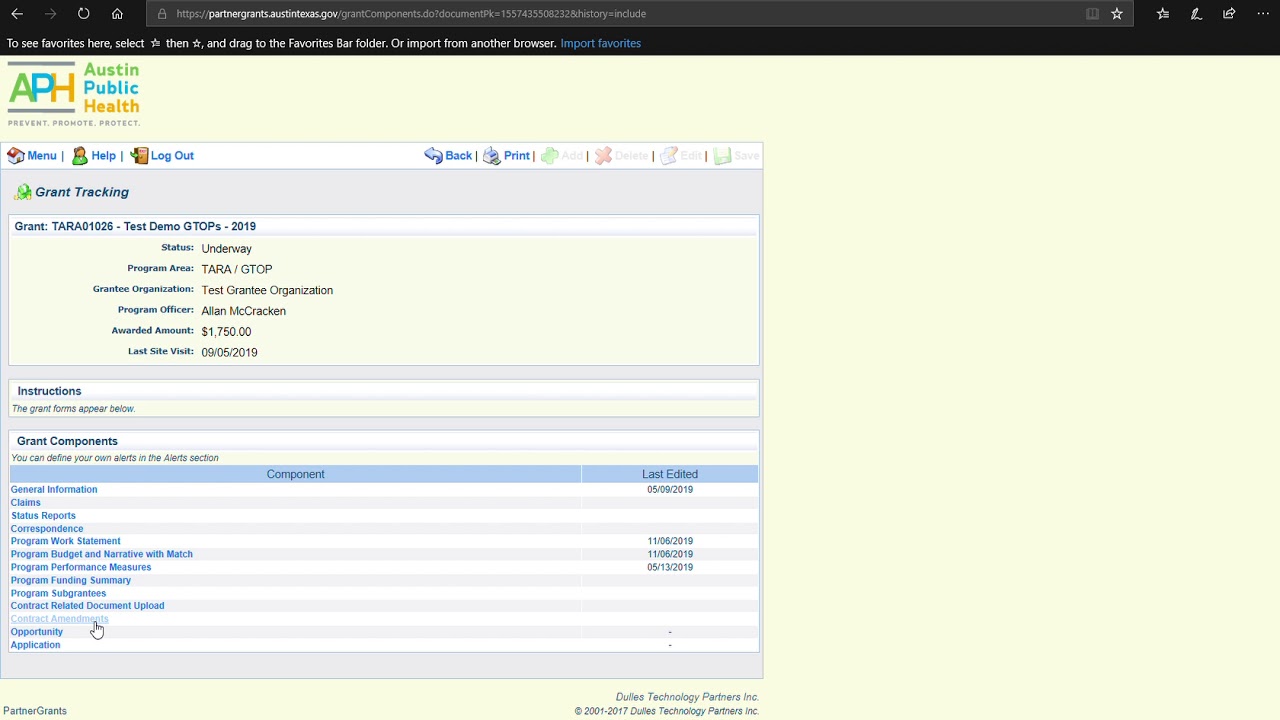A horizontal screenshot of a computer screen, likely taken from a desktop or laptop, featuring a predominantly beige-cream colored background with a black rectangular toolbar running across the top. On the upper left, navigation arrows are visible alongside buttons for refreshing and returning to the home page. The center of the toolbar contains the address bar with the URL "partnergrants.austintexas.gov." Icons for various functions are aligned on the right side of the toolbar.

Just below, there is a prompt indicating, "To see favorites here, select the star, then drag to the Favorites Bar folder or import from another browser," accentuated by an "Import Favorites" link in blue. Further down, the header reads "APH, Austin Public Health - Prevent, Promote, Protect," providing options for "Menu," "Help," "Log out," "Back," and "Print."

The website focuses on grant tracking, presenting fields for "Grant name," "Test Demo," "Status," "Program area," "Grantee organization," "Program officer," "Awarded amount," and "Last site visit." It also offers sections under "Instructions" and "Grant Components," which include clickable blue links for "General Information," "Claims," and "Status Reports," among others. The bottom of the page credits Dualist Technology Partners Incorporated and includes copyright information.